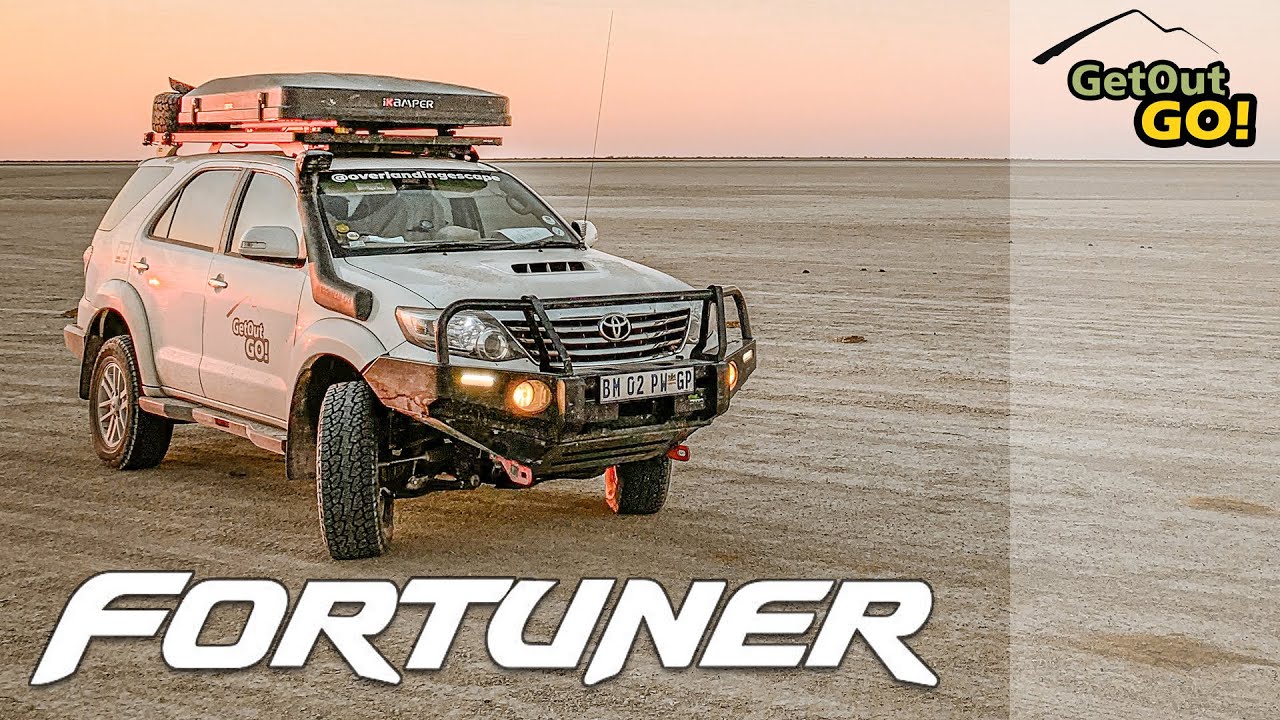The image is a horizontally oriented advertisement featuring a white Toyota Fortuner SUV in a desert landscape, viewed from a three-quarter front-side angle. The vehicle sits on a sandy plain at dusk, with the last rays of sunlight coming from the left, casting a pinkish hue across the sky. The SUV, equipped with four doors, a large black front grille, a protective bar, and smaller tires turned towards the front, features various accessories. On its roof, there's a black rack that includes a storage container, a spare tire, and a pop-up tent. It also has a snorkel for the exhaust.

At the top of the image, there is text in green and yellow letters saying "Get Out Go!" accompanied by an illustrated mountain outline. Below the vehicle, large white text reads "Fortuner." The right side of the image has a slightly faded section, enhancing the desert's vast emptiness, and the vehicle appears unoccupied, emphasizing its readiness for adventure. This intricate composition highlights the rugged yet stylish design of the Toyota Fortuner, inviting viewers to embark on their own outdoor escapades.